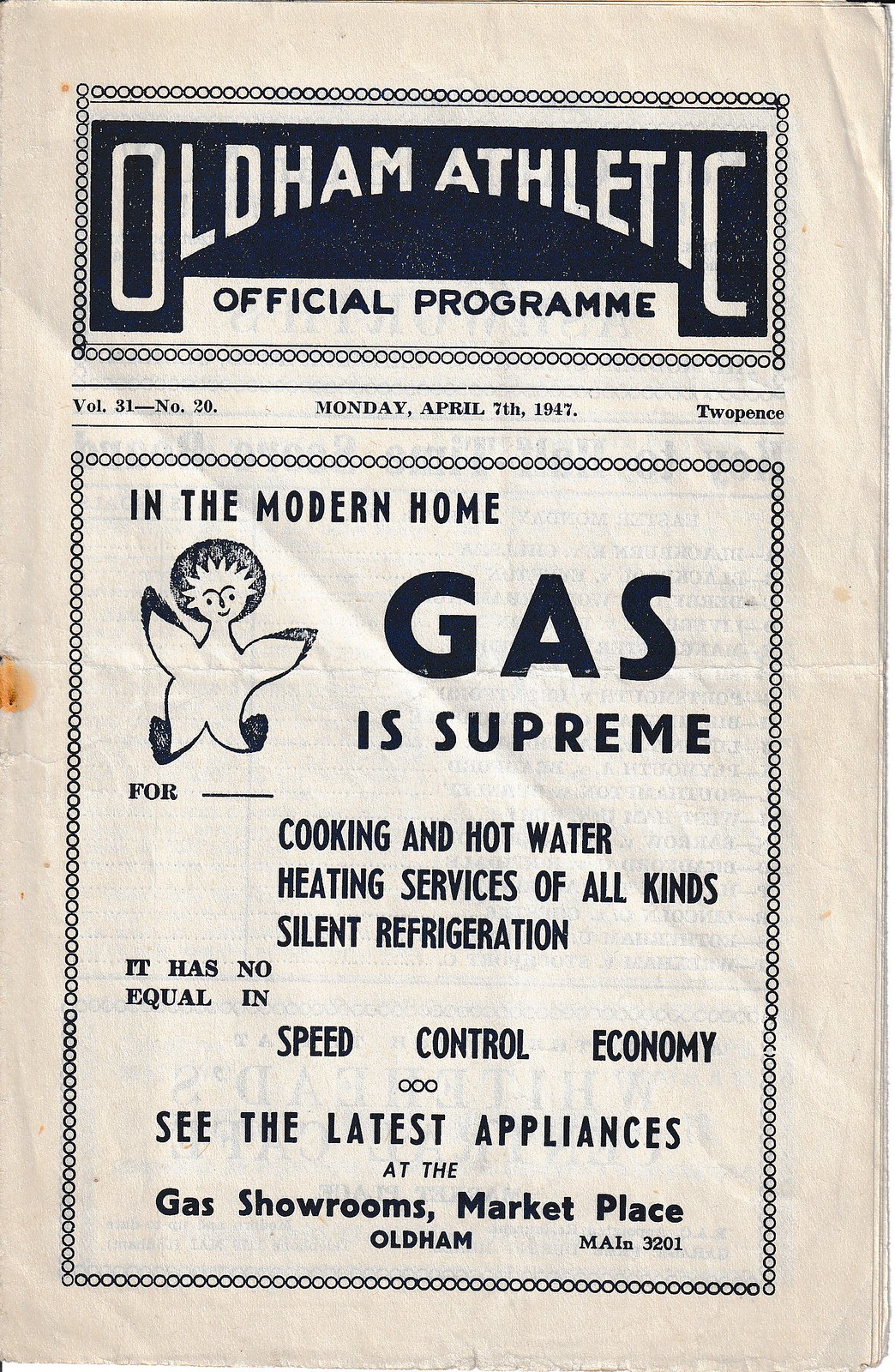The image depicts a vintage, wrinkled, and creased program for a sports team, specifically "Oldham Athletic," dated Monday, April 7th, 1947. The cover has a paper texture and a tannish-yellow color, featuring a prominent black rectangle at the top with the text "Oldham Athletic" in white font. Below it, a white rectangle with black text reads "Official Program." Additionally, the header includes details such as "Volume 31, Number 20" and the price, "Two Pence." The central portion of the image is occupied by an advertisement with a black circle-bordered frame, stating "In the modern home, gas is supreme." It promotes various services, including cooking, hot water heating, and silent refrigeration, emphasizing their speed, control, and economy. The ad also encourages viewers to visit the latest appliances at the gas showrooms in the marketplace, provided with the contact detail "MAIN 3201." The program also bears a distinctive logo featuring a plant and the sun, adding a unique touch to this historical document. Notably, there is visible wear, with multiple creases and a stain on the upper right corner and middle left area, respectively.